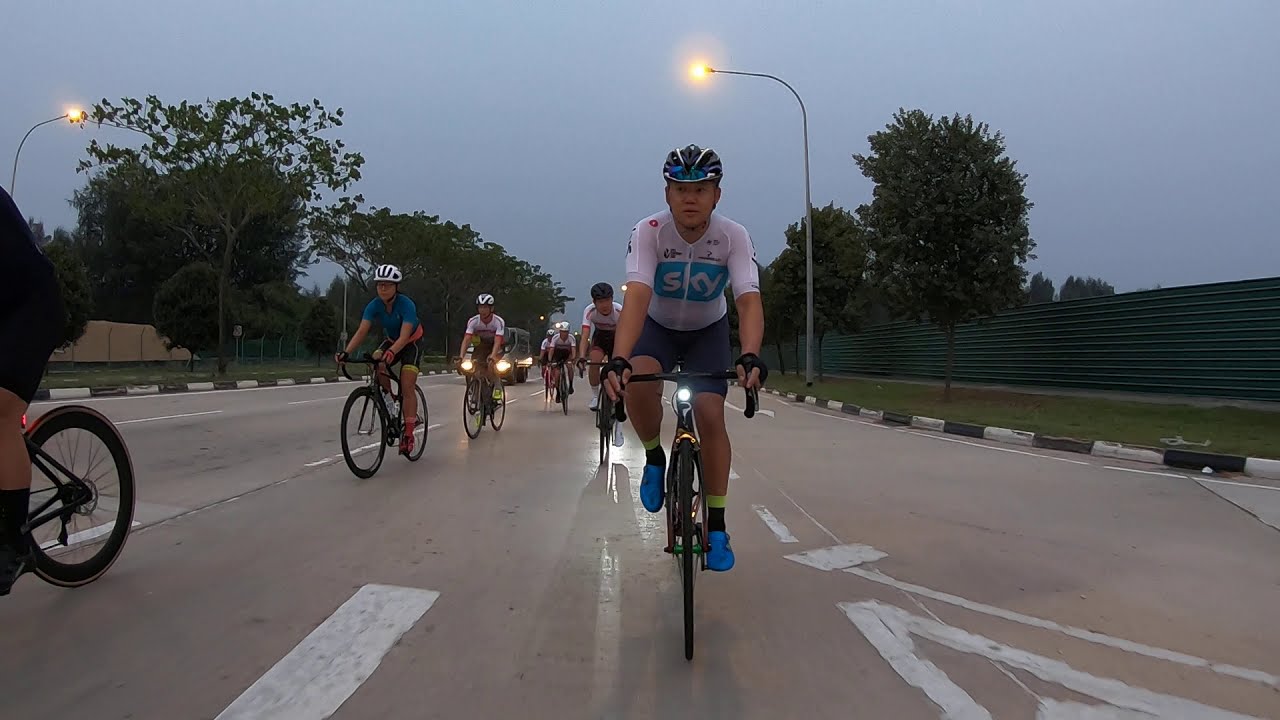The image depicts a group of cyclists participating in what appears to be a race or organized ride, taking place either at dusk or early morning under an overcast sky. The scene is predominantly gray with a multi-lane, smoothly paved road of a grayish-purple hue featuring white markings. Street lamps are illuminated, hinting at the low light conditions. 

At the forefront, there is an Asian man wearing a white jersey with a blue logo that reads "Sky." His attire includes a blue, black, and white helmet, blue riding shoes, blue riding shorts, black gloves, and he has a headlight mounted on his black bicycle, which features a P logo. His blue sneakers are complemented by black and yellow socks. Behind him are multiple cyclists similarly dressed in tight-fitting riding gear, helmets, and cycling shoes, forming two lines going towards the camera. On the far left, the rear wheel and the left leg of another rider are partially visible.

In the background, to the left side of the image, the road curves diagonally, while to the right, there’s a curbside lined with trees, a fence wall, and a light pole. Additionally, a vehicle follows the cyclists further down the road. The atmosphere and elements suggest a synchronized event in progress amidst a serene, cloudy setting.